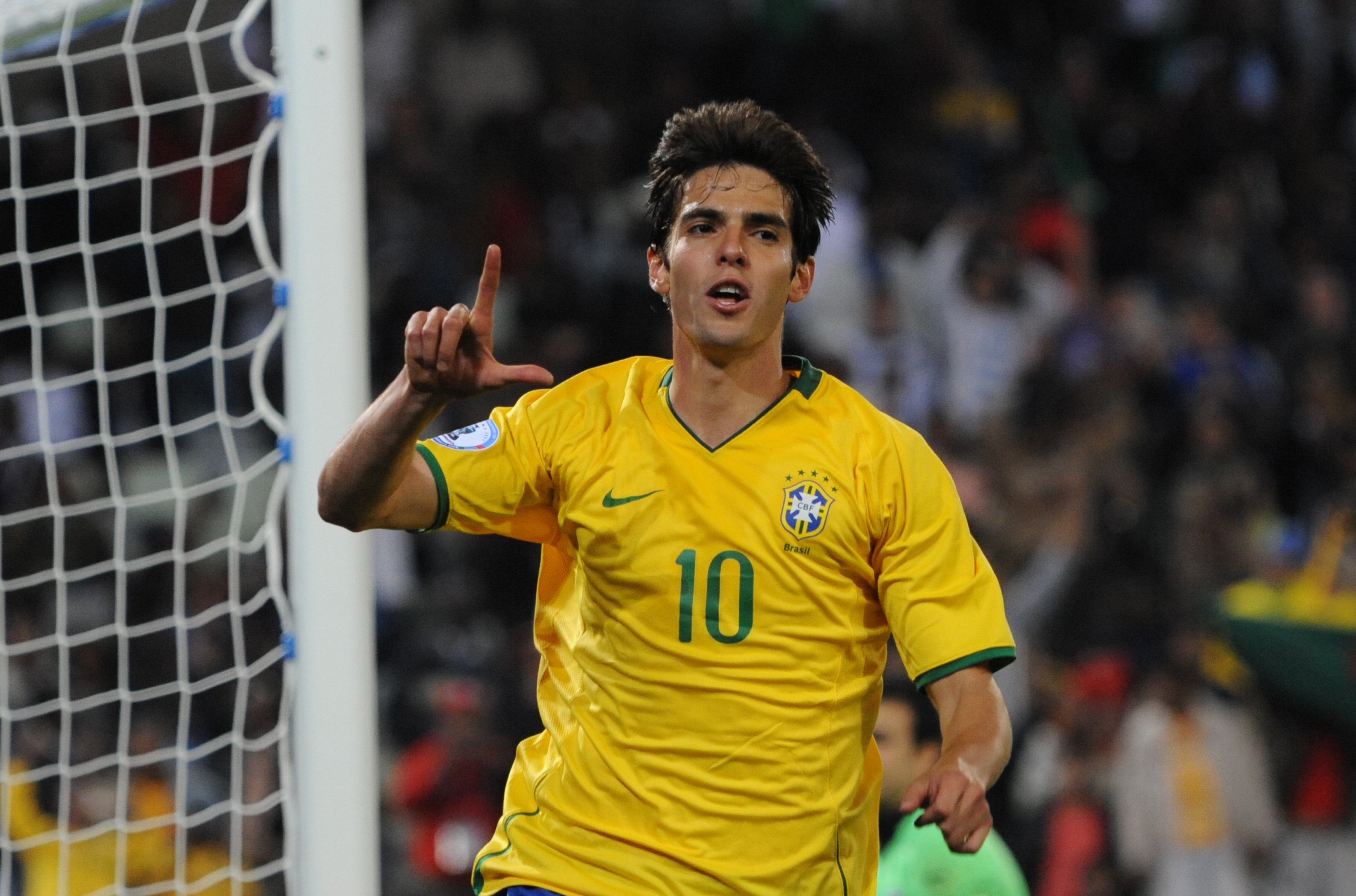In this vivid image, a young male soccer player is captured mid-action during a live event. He is seen running, his sweat glistening under the stadium lights. He has short brown hair, styled in a way that makes it appear full and slightly tousled. The player is clad in a bright yellow jersey adorned with a green Nike swoosh on the right side of his chest, the number 10 prominently displayed in green in the middle, and additional details in blue and white. The collar and sleeve ends of the jersey are also green. 

The player's right hand is raised, forming an 'L' shape with his index finger and thumb, while his other hand naturally rests by his waist. To the left of him is a white soccer goal with a thick pole and white netting, clearly visible in the scene. In the background, though blurred, a colorful crowd in the stands adds to the electric atmosphere, showcasing a mix of white, red, blue, green, and yellow hues amidst a darker backdrop. An official in a green jersey is also discernible on the field, contributing to the on-field activity and vibrancy of this dynamic soccer event.